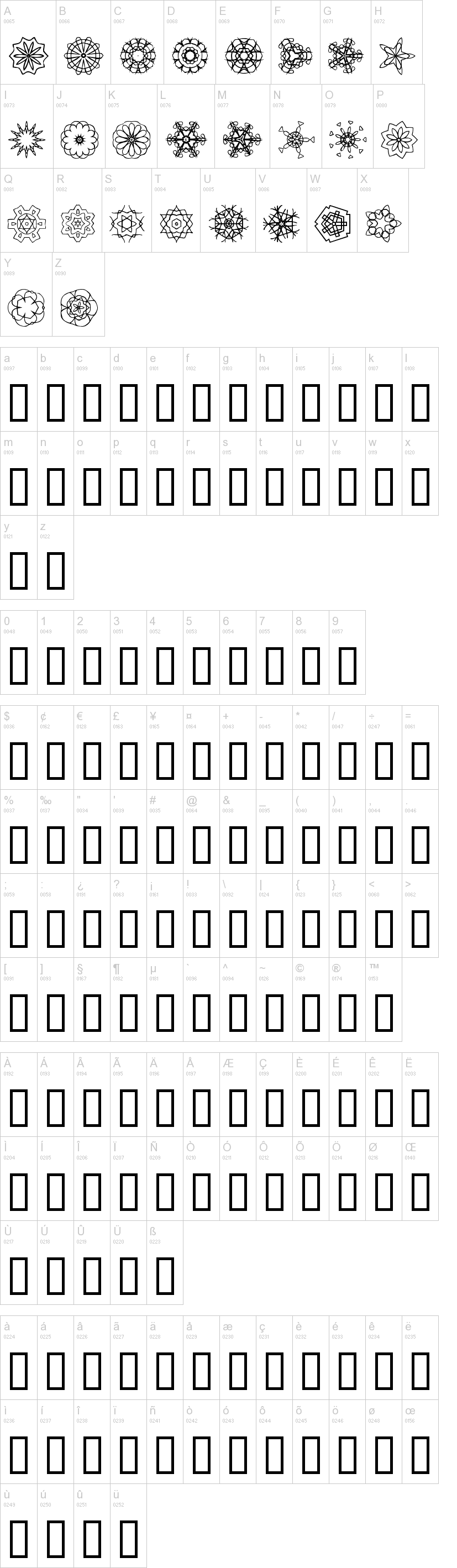The image depicts a comprehensive grid of alphanumeric characters and symbols, each assigned a unique code and adorned with intricate designs. Starting from the top left, the characters appear in sequential order beginning with uppercase 'A' at position 0065, which resembles a snowflake. 'B', marked as 0066, also emulates a snowflake but is surrounded by a circle. The grid continues in this pattern, listing letters from A to Z with each letter on subsequent lines—A to H on the first line, I to P on the second, Q to X on the third, and Y to Z on the final line.

Beneath the uppercase letters, the grid transitions to lowercase letters, each characterized by a rectangle embedded within them. Following this, the grid features numerals from 1 to 9, also encased in rectangular forms. 

At the bottom of the image, the layout expands to include symbols and various stylistic variations of the letter 'A', filling the entirety of the area. Notably, the letter 'U' is accompanied by a specific code and similarly incorporates a rectangle within its design, suggesting a card-like motif that pervades the entire image, imparting an organized and artistic structure to the alphanumeric and symbolic elements displayed.